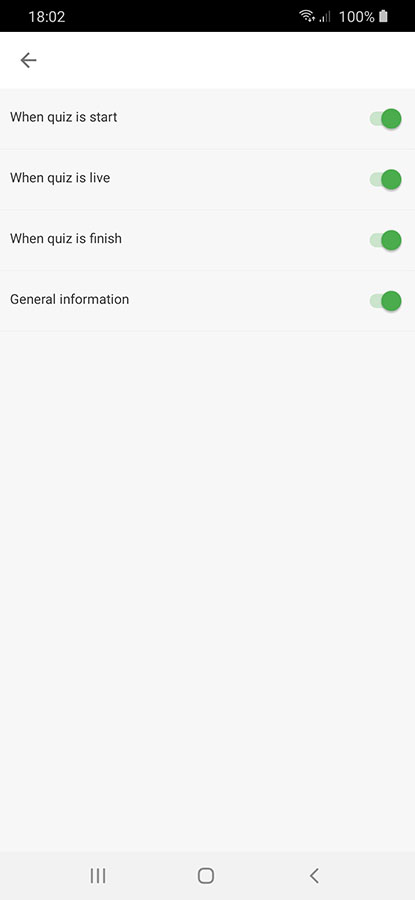The image appears to be a screenshot of a mobile device, identifiable by its aspect ratio and the presence of a status bar at the top. The status bar shows the time as 18:02, a fully charged battery at 100%, and a Wi-Fi connection. Just below the status bar is a back button, represented by a left-pointing arrow.

The main content consists of four lines of black text, each accompanied by a green toggle icon, which suggests that these options are currently enabled. The first three lines read as follows: "When quiz is start," "When quiz is live," and "When quiz is finish." These lines likely correspond to notifications for different stages of a quiz. The fourth line, "General information," likely pertains to general notifications.

The background of the image is primarily light gray, providing a neutral backdrop that highlights the black text and green toggles. The overall design appears simple and straightforward, focusing on user interactions with the toggles to manage quiz-related alerts.